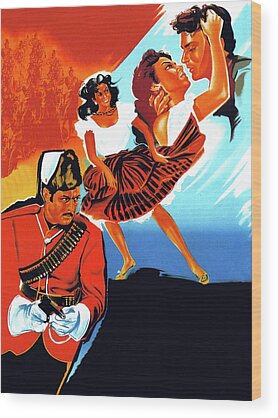The painting, reminiscent of a dramatic movie poster but devoid of any text, appears to be done in acrylic on canvas. It is a composition replete with vivid and contrasting imagery. In the bottom left corner stands a stern-looking man dressed in a red military jacket adorned with black lines down the sleeves. He sports white gloves and a black and white hat, with a bandolier of ammunition slung across his chest. He holds a small pistol in his hand and gazes angrily toward the lower right.

Directly above him and slightly to the right, the painting features a woman with very dark black hair, appearing to dance. She's dressed in a white blouse and a reddish-brown skirt and is possibly wearing high-heeled shoes. Her dynamic pose suggests motion, as if captured mid-dance.

Dominating the top right of the canvas, another scene unfolds: a couple on the verge of a kiss. The man, situated at the very top right, has his hand gently placed around the back of the woman's neck. The woman, whose face is partially visible from the side, has her hand in the man's hair, pulling them closer together. Their lips are mere inches apart, adding a sense of intimate tension.

The background of the painting is a blend of contrasting colors. The top left is saturated with reds, resembling a burning forest, adding a sense of chaotic urgency. The bottom right fades into dark, almost black hues, emphasizing the foreboding atmosphere. The middle section features blue tones, creating a stark contrast with the surrounding colors and tying together the various elements and characters within the painting.